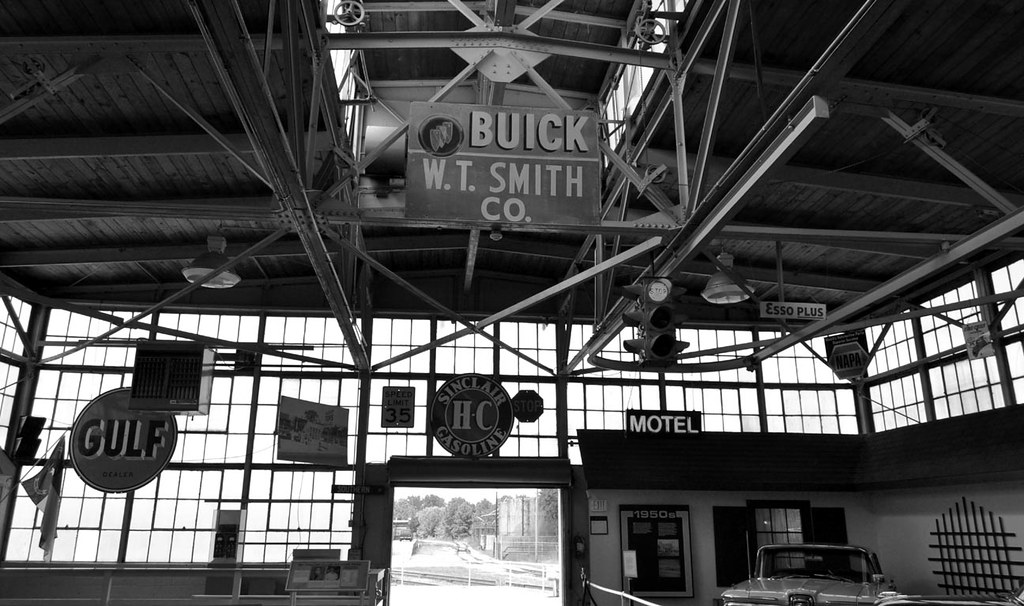This detailed black-and-white photograph showcases an indoor vintage car factory or garage, brimming with historical charm and signage. Dominating the scene is a prominent sign that reads "Buick W.T. Smith Company," suspended above the wooden roof braced by girders. The surrounding walls are lined with numerous tall windows, which flood the space with natural light. Hanging from the ceiling are various other signs, including "Gulf," "Sinclair H.C. Gasoline," "Motel," and "S.O. Plus," as well as functional light fixtures and even a traffic stoplight. 

In the lower part of the photo, partly cut off, sits a classic car from the 1950s, parked near what appears to be a mock motel entrance, adding an intriguing layer to the scene. At the center bottom, an open doorway suggests a space bustling with activity, possibly where cars once came in and out. This image captures not only the essence of a bygone era in automotive history but also the intricate details of a working car garage with its eclectic mix of industrial and retro elements.